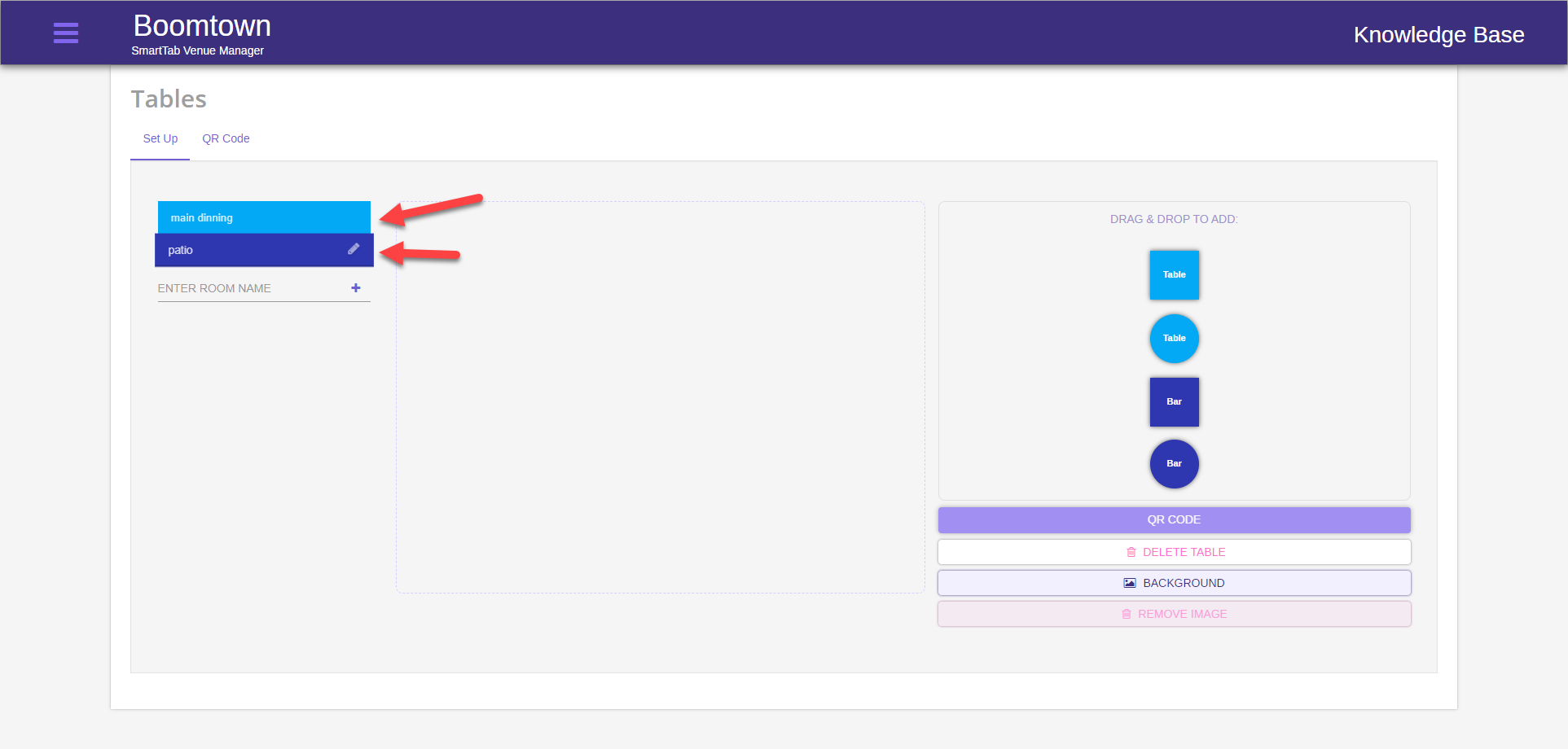Screenshot of Boomtown's SmartTab Venue Manager interface: 

The top section features a blue box with the text "Boomtown's SmartTab Venue Manager." On the right-hand side, there's a "Knowledge Base" section. The primary background is white, showcasing table setup options and a QR code area.

In the middle section, a gray background indicates different dining areas. The "Main Dining" area is highlighted in an aqua box with a red arrow pointing to it. Adjacent to this, a dark blue box labeled "Patio" is also marked with a red arrow.

Beneath these sections, there's an "Enter Name" input field. The interface allows for drag-and-drop table arrangement. Two types of tables, square and round, are displayed in teal. Additionally, there are two types of bars, round and square, shown in dark blue. A QR code bar is highlighted in lavender. The option to delete tables is presented in white.

The background continues in gray, with a pink box labeled "Remove Image." The overall interface provides a comprehensive and detailed table setup and management system for venue spaces.